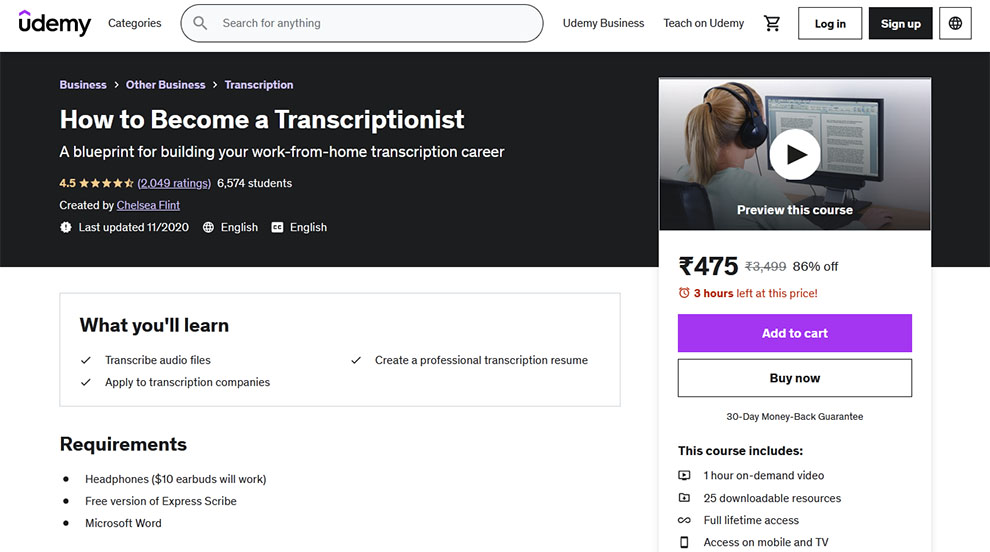The image is an advertisement for Udemy, featuring a course on building a work-from-home transcription career. The image has a white background that blends seamlessly into the Udemy platform's prolific interface. In the upper left-hand corner, the Udemy logo is prominently displayed, followed by navigation options such as "Udemy Business," "Teach on Udemy," "Shopping Cart," "Log In," "Sign Up," and a global icon for language or location settings. 

A black rectangle situated below the main navigation bar highlights an ad for the course "How to Become a Transcriptionist: A Blueprint for Building Your Work-From-Home Career." This course boasts a rating of 4.5 stars and has been attended by 6,574 students. It is created by Chelsea Flint. Potential students are given the option to preview the course or purchase it for 475 rupees, with the caveat that the price is 86% off for the next three hours.

The ad further details what the course entails, promising to teach students how to transcribe audio files, apply to transcription companies, and create a professional transcription resume. Requirements for the course include having a pair of headphones, a free version of Express Scribe software, and Microsoft Word. Additionally, the right side of the advertisement lists what the course includes, providing comprehensive insight into the offerings for prospective students.